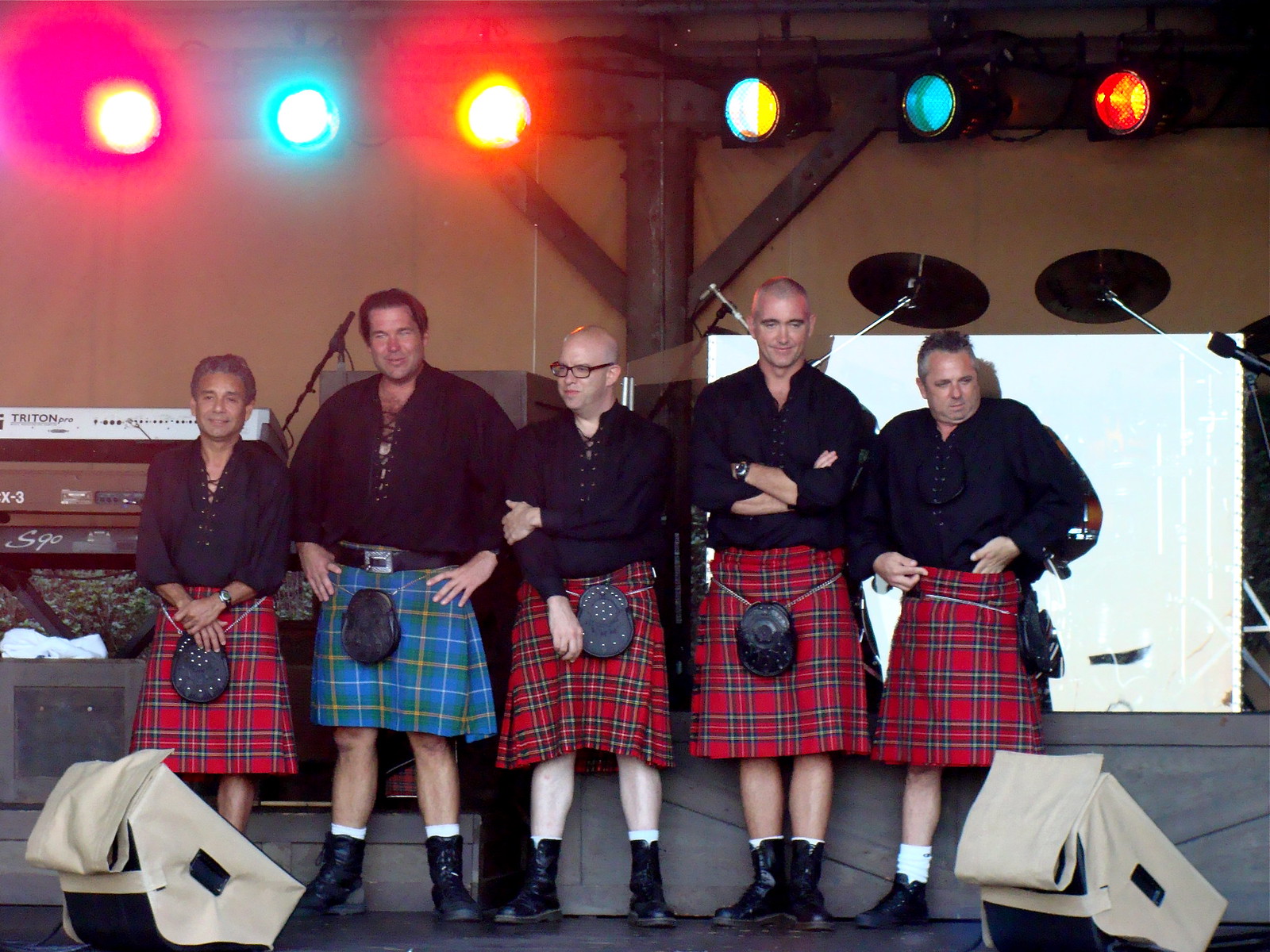In this vibrant color photograph taken indoors, five men stand on a performance stage, each adorned in traditional Scottish attire. Four of the men are dressed in striking red tartan kilts, while the man second from the left stands out in a blue kilt with yellow, white, and green stripes. Each kilt is complemented by a black sporran pouch, neatly positioned at the front. They uniformly wear all-black, long-sleeved, lace-up shirts, shin-length black boots, and most exhibit white socks above their boots, though the feet of the man on the far left are out of view.

In the background, a dynamic array of spotlights, strung in a horizontal row, cast a colorful brilliance: hues of pink, blue, turquoise, red, yellow, and orange illuminate the scene, with some flaring slightly into the camera on the left side. These lights create a vibrant atmosphere, hinting at an energetic musical performance. The presence of a microphone stand, the edge of a keyboard, and the shiny cymbals of a drum kit partially obscured to the right further emphasize the performance setting. Additionally, the backs of speakers with light tan canvas covers are visible in the left and right foreground, completing the stage ensemble.